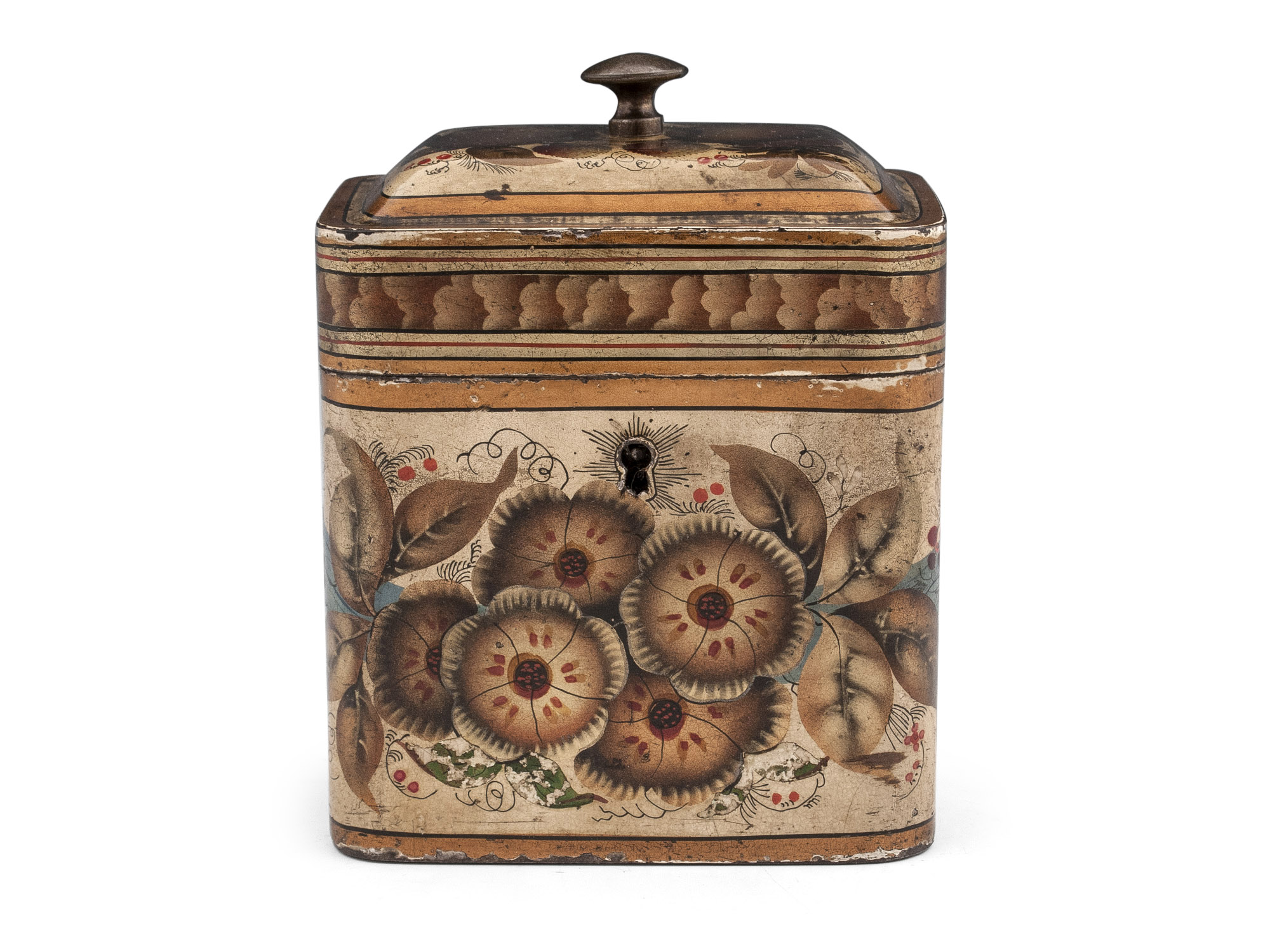The image depicts an old, aged tin container set against a white background. The tin is adorned with a faded floral design featuring brown poppies with white edges and browned leaves, hinting at its age and wear. The container has a rustic appearance with areas where the paint has been rubbed off over time, revealing a misty brown edge that transitions into weathered stripes of red, white, and golden hues. The front of the tin has a keyhole, suggesting it might have once been lockable. Atop the container sits a lid with a small silver knob, which one would use to remove the lid. The base of the tin shows signs of further decay, with paper peeling off, exposing the oxidized, grayish-white background underneath.